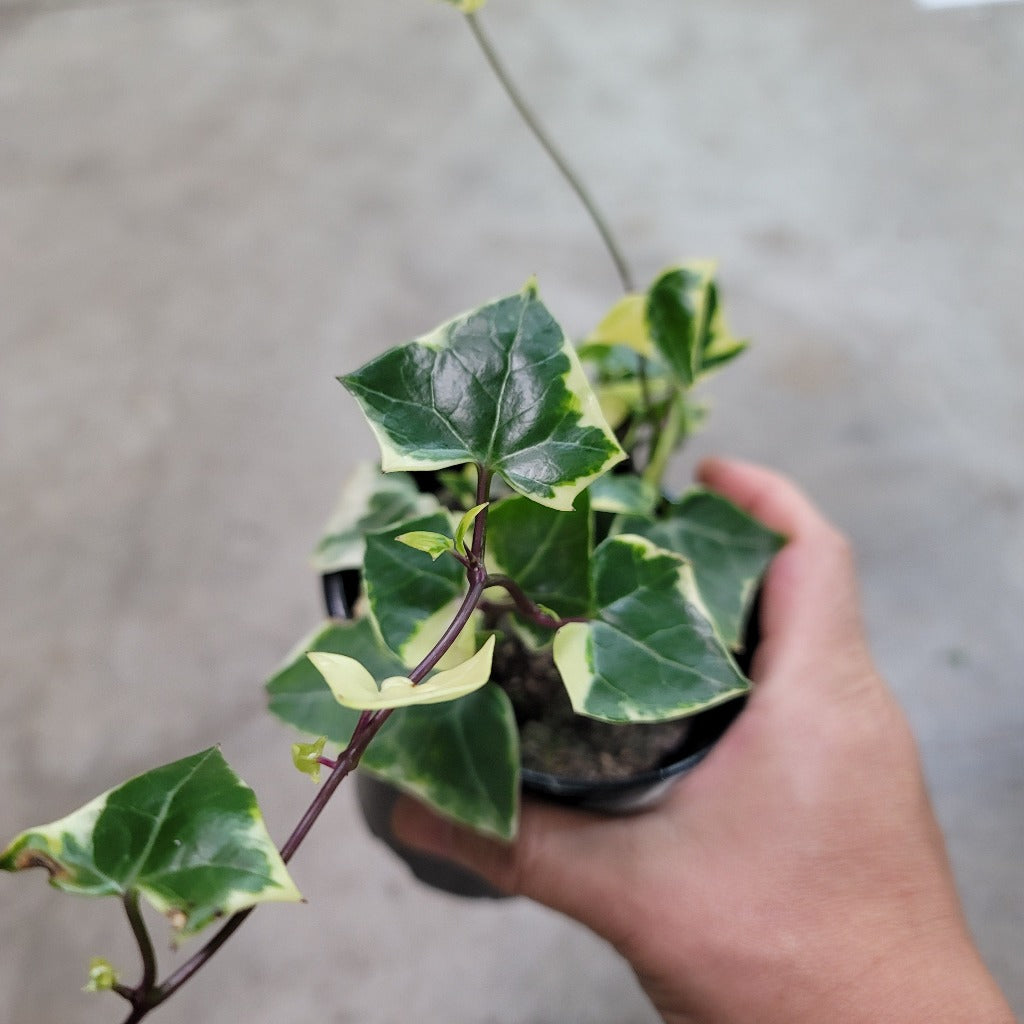In the photograph, a person is holding a small plant pot, painted black, in their right hand. The background features a grey surface, likely the ground, slightly blurred to draw focus to the plant. The plant itself has intriguing foliage: its purple stems support leaves that are dark green in the center with light green edges. Some newer leaves are just starting to emerge. The plant appears small, and though it has some realistic elements like visible dirt, the purple stems give it a somewhat artificial appearance. Daylight illuminates the scene, ensuring the entire plant and pot are clearly visible.